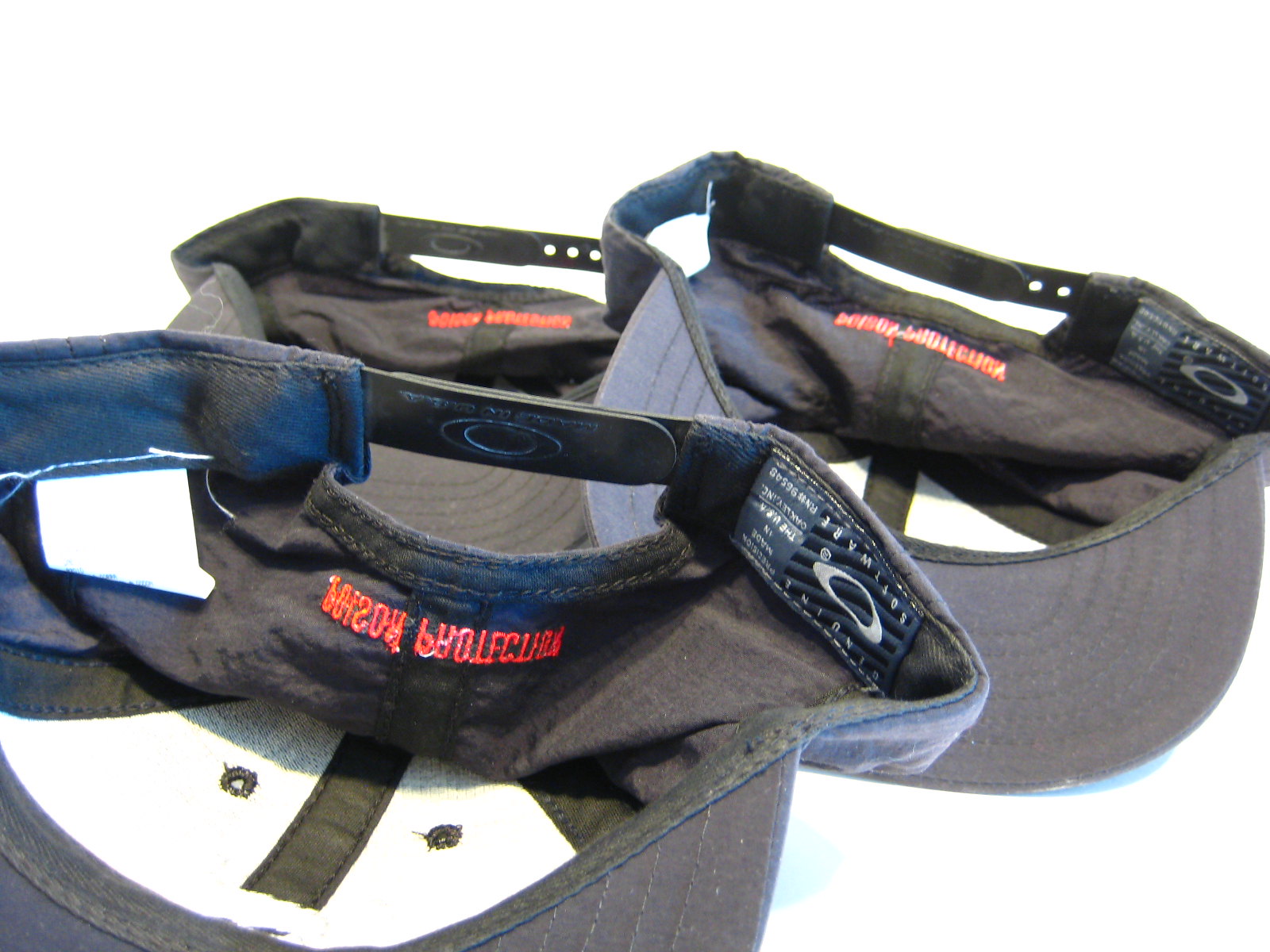This up-close studio photograph features three clean snapback baseball caps, presented against a plain white background. The caps are positioned upside down, showcasing their interiors as well as the bottom portions of their bills. Two of the caps are a light blue-gray color, while the third is dark gray. Each hat has an embroidered text stitched in red along the back, however, the lettering is difficult to decipher due to its upside-down and backwards orientation. Inside the hats, various tags are visible, including brand tags and adjustable components used to fit the hats to different head sizes. Black lining and black bills contrast with the overall navy-blue color scheme of the hats, adding to their detailed design elements.